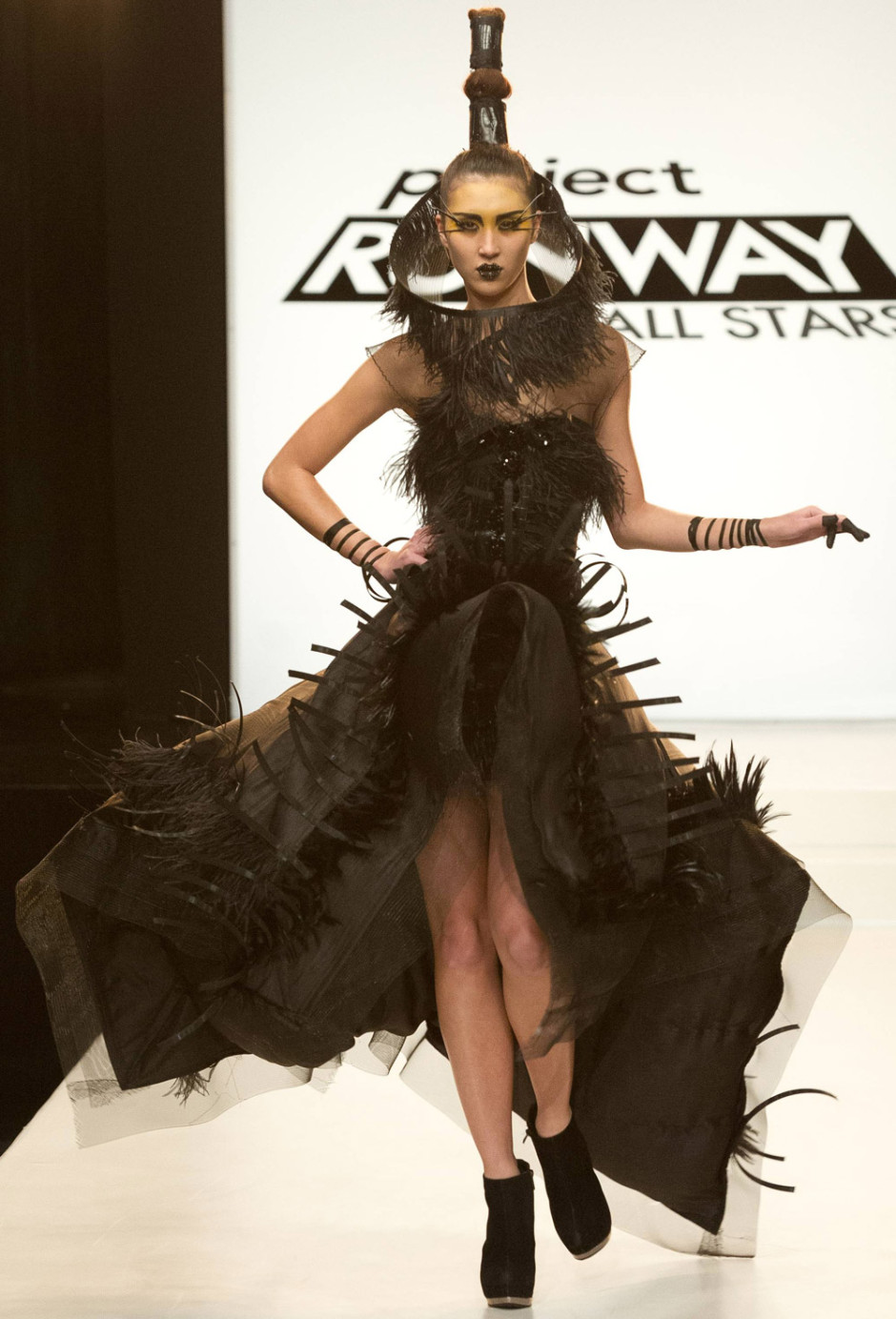In this close-up photograph of a model striding down a beige runway at Project Runway All-Stars, her striking dark brown and light brown dress captures the eye. The intricately designed dress flows dramatically out to the sides, allowing glimpses of her legs. It features frills starting near the hip area and extending down where it fans out. The bodice of the dress appears almost fur-like, accented with four prominent black balls situated just below her chest. Her light-complected arms are adorned with a multitude of tight black or brown bracelets—five on the left and seven or eight on the right. The fingers on her right hand are notably brown. Complementing her ensemble are dark shoes, likely black booties, that are cut off just at her heels. Her hair is pulled back into a ponytail and is adorned with a large, ornate brown headpiece that juts vertically behind her head. Her accessories include a brown, fur-lined or feathered veil. The background, though partially obscured, clearly indicates the setting with the "Project Runway All-Stars" logo behind her, featuring "Project" and "All-Stars" in black and "Runway" in white text within a black rectangle. A black curtain to her left adds to the dramatic ambiance of the scene.